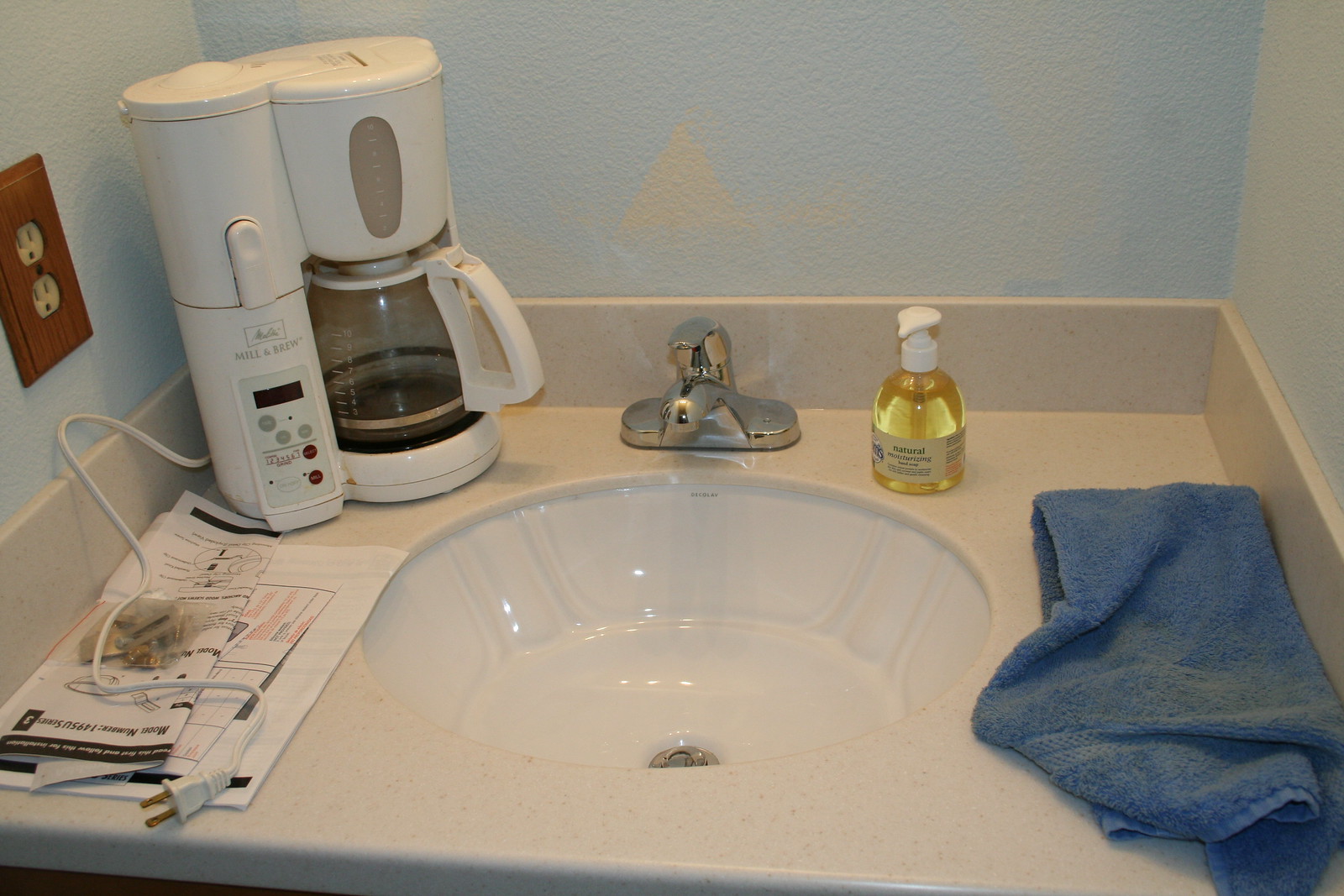This photograph captures a sink area in what appears to be a budget hotel room, characterized by its subpar condition. The sink is set into a plastic countertop designed to mimic beige faux granite, possibly Corian, and the matching backsplash shares this faux finish. The sink itself is a white, fluted design, paired with a chrome faucet. A bottle of yellow liquid hand soap is present, dispensing soap via a pump.

Adjacent to the sink, there is a visibly dirty blue towel. A coffee maker, which is not plugged in, sits on the countertop; its kettle section is heavily stained, likely due to extensive use. The walls show a haphazard paint job, with the left wall painted blue, the side wall on the right painted tan, and the back wall displaying a botched mix of blue and tan. Lastly, there is an electrical outlet with a wooden cover over the sockets, adding to the room's overall neglected appearance.